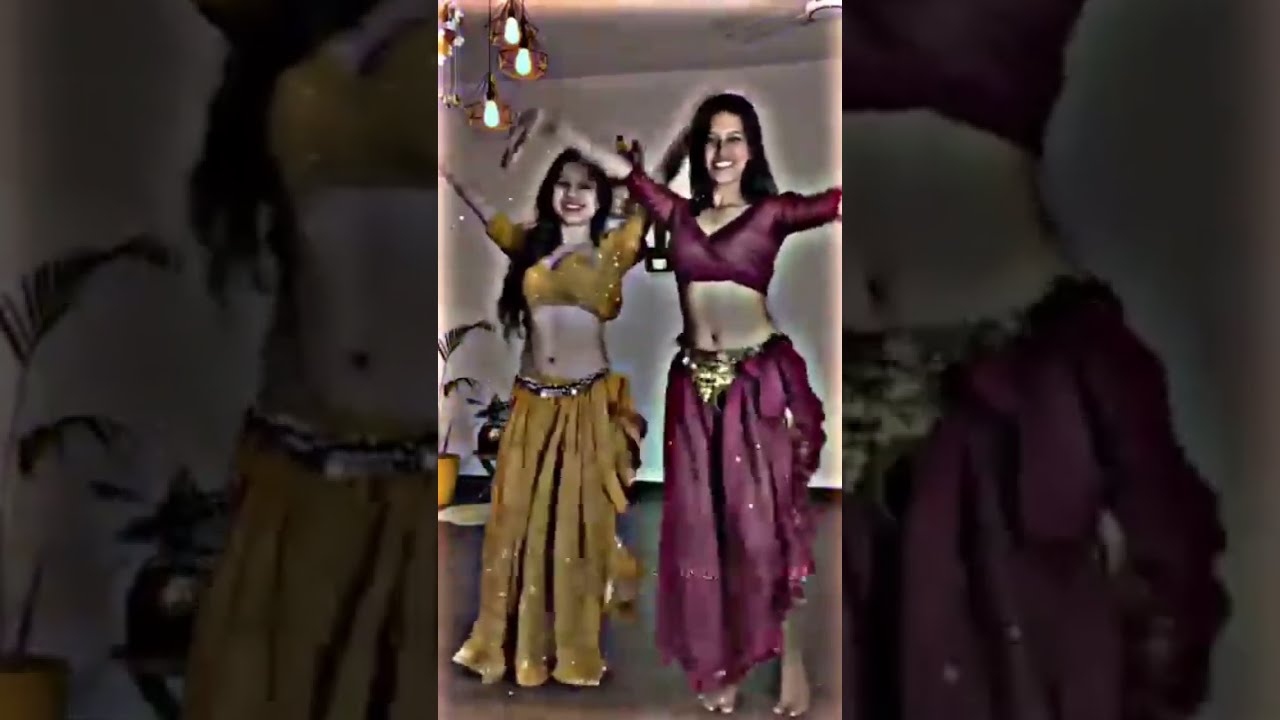The image is a lively scene capturing two women, who appear to be Indian, engaged in belly dancing. Both women have long black hair and are smiling directly at the camera, indicating they are aware of being photographed. They exhibit ornate, long-sleeved dancing outfits that expose their bellies. The woman on the left is dressed in a goldish-yellow outfit adorned with sparkles, while the woman on the right dons a purplish outfit with a skirt that complements her top. They are barefoot and accompanied by minimal yet detailed accessories, including gold belts, with the belt on the right being more elaborate.

The setting is an open room with white walls and a brown floor. Adorning the upper left are white dangling lights with gold trim. A potted plant is visible behind the woman in the yellow outfit. The picture is a screenshot from a portrait video and shows an altered effect, reflected by the filtered and heavily modified appearance of the dancers. Additional elements from the video include darker, zoomed-in images on either side of the main photo, focusing on their midsections but with lower lighting, showcasing details of their vibrant costumes and the lively energy of their dance moves.